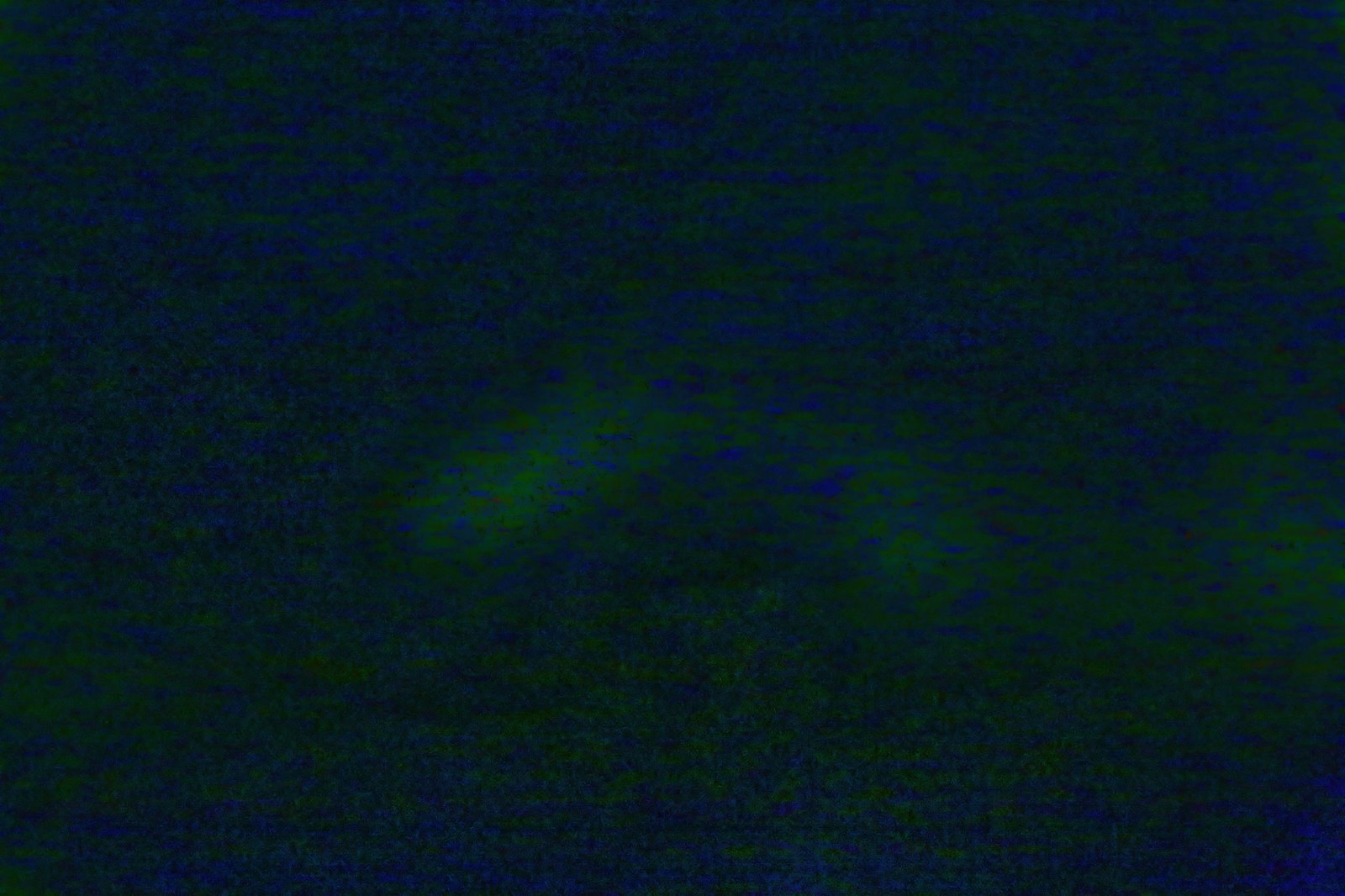The image is very blurry and grainy, resembling a photo taken by a low-quality night vision camera or an exterior security camera during the night. Predominantly dark in color, the picture features a mix of dark green, light green, and various shades of blue, creating an almost eerie atmosphere akin to a scene from a horror movie. The central area of the image is brighter, with light green tones, possibly hinting at the vague outline of a frowning, round face, shrouded in shadows. Surrounding the center are numerous dark blue and green spots, all closely clustered together, adding to the overall sense of ambiguity and mystery. Despite the effort to discern details, the scene remains largely inscrutable, evoking the experience of checking a security app that alerts to motion but reveals an indecipherable, low-quality, and almost completely dark image.